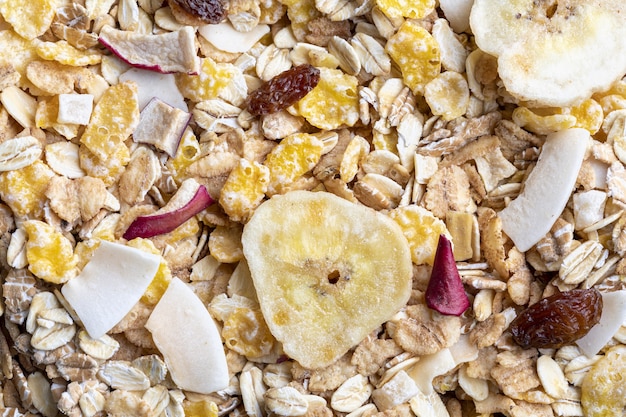This vibrant close-up photograph showcases a diverse and textured mix of granola. Dominating the image are a variety of dried fruits and grains, including noticeable slices of dried bananas, coconut flakes, and pieces of pineapple and mango. Interspersed throughout are dried grapes, red onion slices, and various yellow chunks, which possibly include additional tropical fruits. The granola is also rich with oats, forming the bulk of the mixture. Additionally, the presence of dried cranberries, corn flakes, and possibly corn puffs or amaranth adds more texture and detail to the mix. The bright image, devoid of any external background, invites us into a visually appealing and nutritious breakfast snack, bursting with flavor and wholesome ingredients.